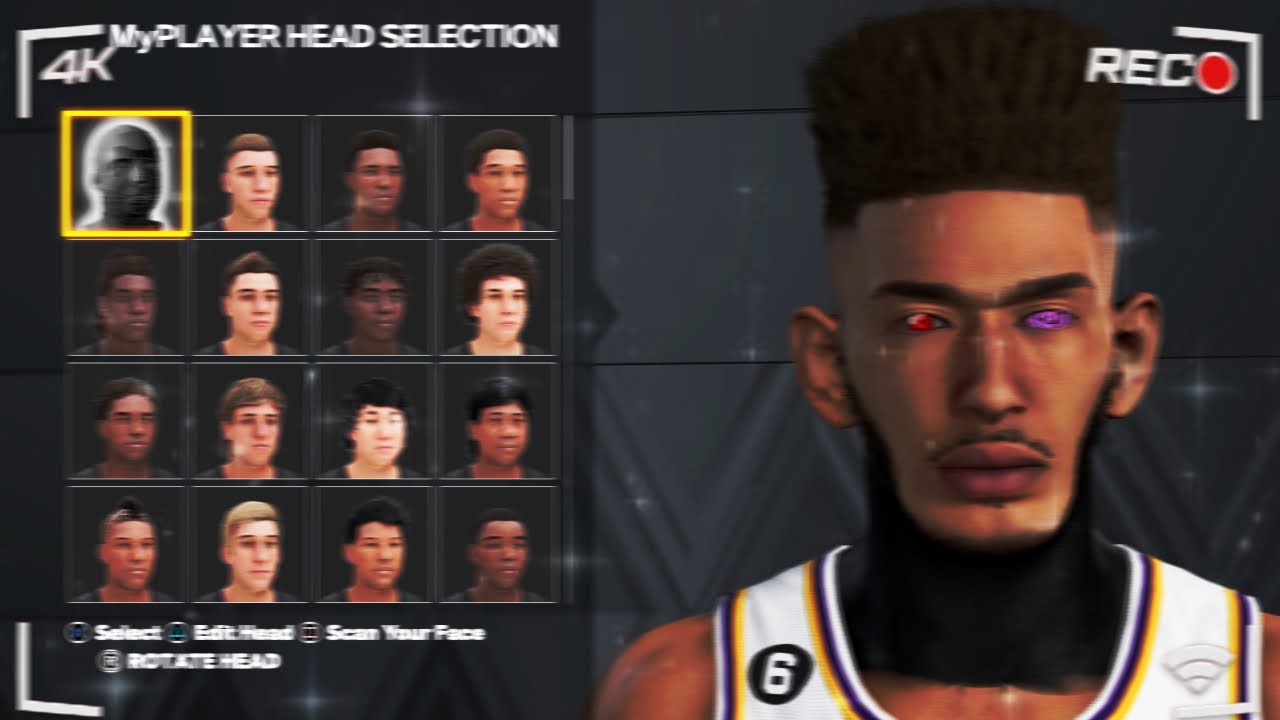This screenshot appears to be from a character selection or customization screen of a video game on a website. The central focus is on a specific character on the right-hand side: a black man with tall, black hair styled distinctively, and a small mustache. His eyes are striking, with an unusual combination of purple and red colors, suggesting an artistic, drawn style. Dressed in a white jersey adorned with yellow and purplish stripes, he bears the number six prominently displayed. 

At the top of the screen, "REC" (possibly indicating 'record') is displayed alongside a red and white circle, which could represent a recording indicator. The left side of the screen is labeled "4k My Player Head Selection." Here, players are presented with a choice of 16 different heads, arranged in four rows of four. Each head represents a different possible character customization option. 

Below these selections, the interface offers various interactive options: "Select," "Edit Head," "Scan Your Face," and "Rotate Head," allowing comprehensive customization of the selected character. The first selection, highlighted in yellow, features an image of a man in black and white, contrasting with the other options, which are in full color. These other selectable heads show a diverse range of male characters of different ethnicities, primarily facing to the right, with various short hairstyles and hair colors.